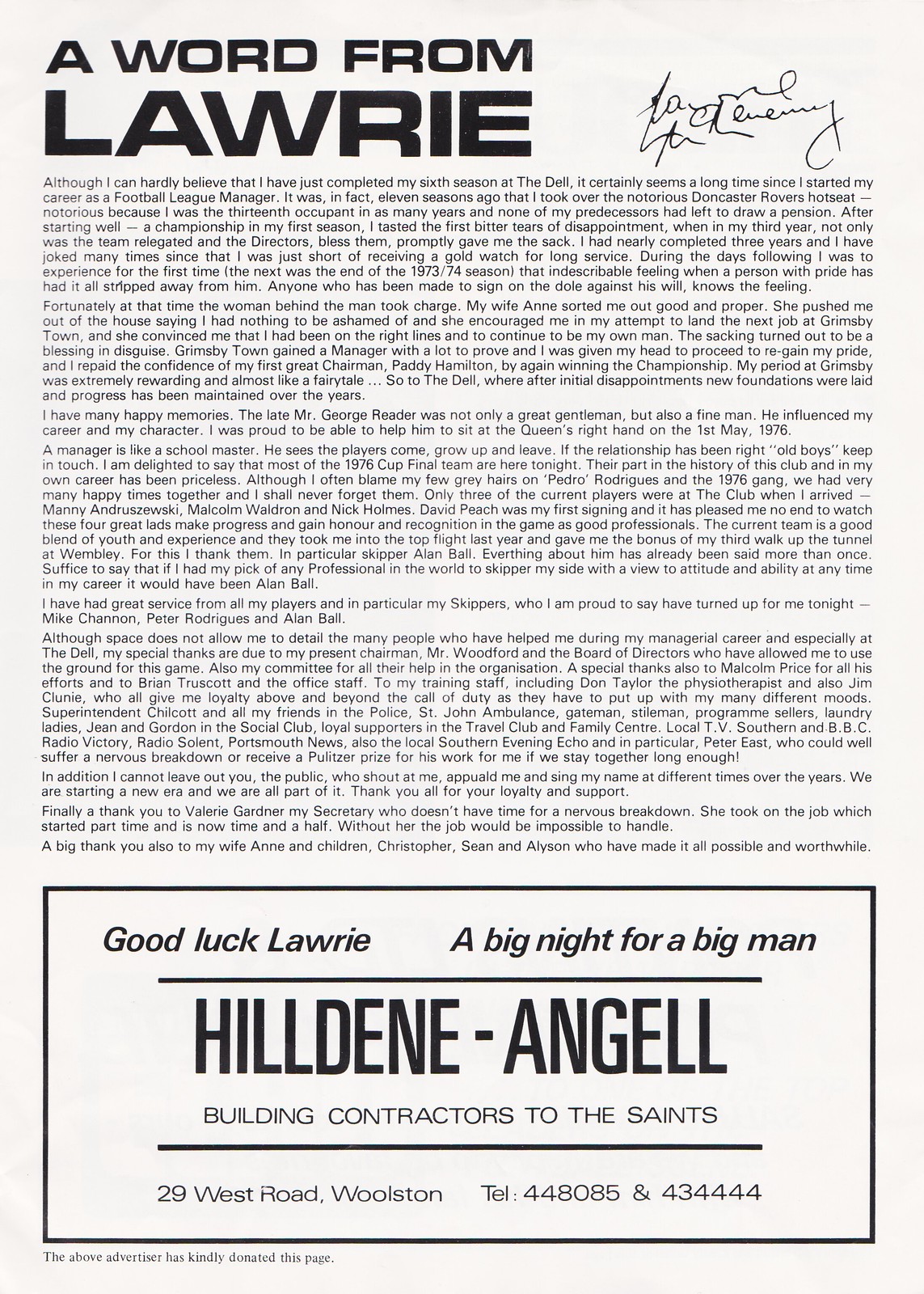The image features a light grey background with black text, presenting a detailed message titled "A Word from Lawrie" positioned in the top left corner. This introductory title is immediately followed by a signature on the top right. The main body of the image contains a densely packed text of 4-5 paragraphs, beginning with the sentence, "Although I can hardly believe that I have just completed my sixth season at The Dell..." This text appears to be a reflective message from Lawrie, a manager of a British football team, directed towards the team and fans, announcing his accomplishments and experiences. Below this message, there is a bordered rectangular section containing an advertisement reading, "Good luck, Lawrie. A big night for a big man," from a business identified as Hill Denny, Angel, building contractors to the Saints, located at 29 West Road, Woolston, with contact numbers 448085 and 434444.